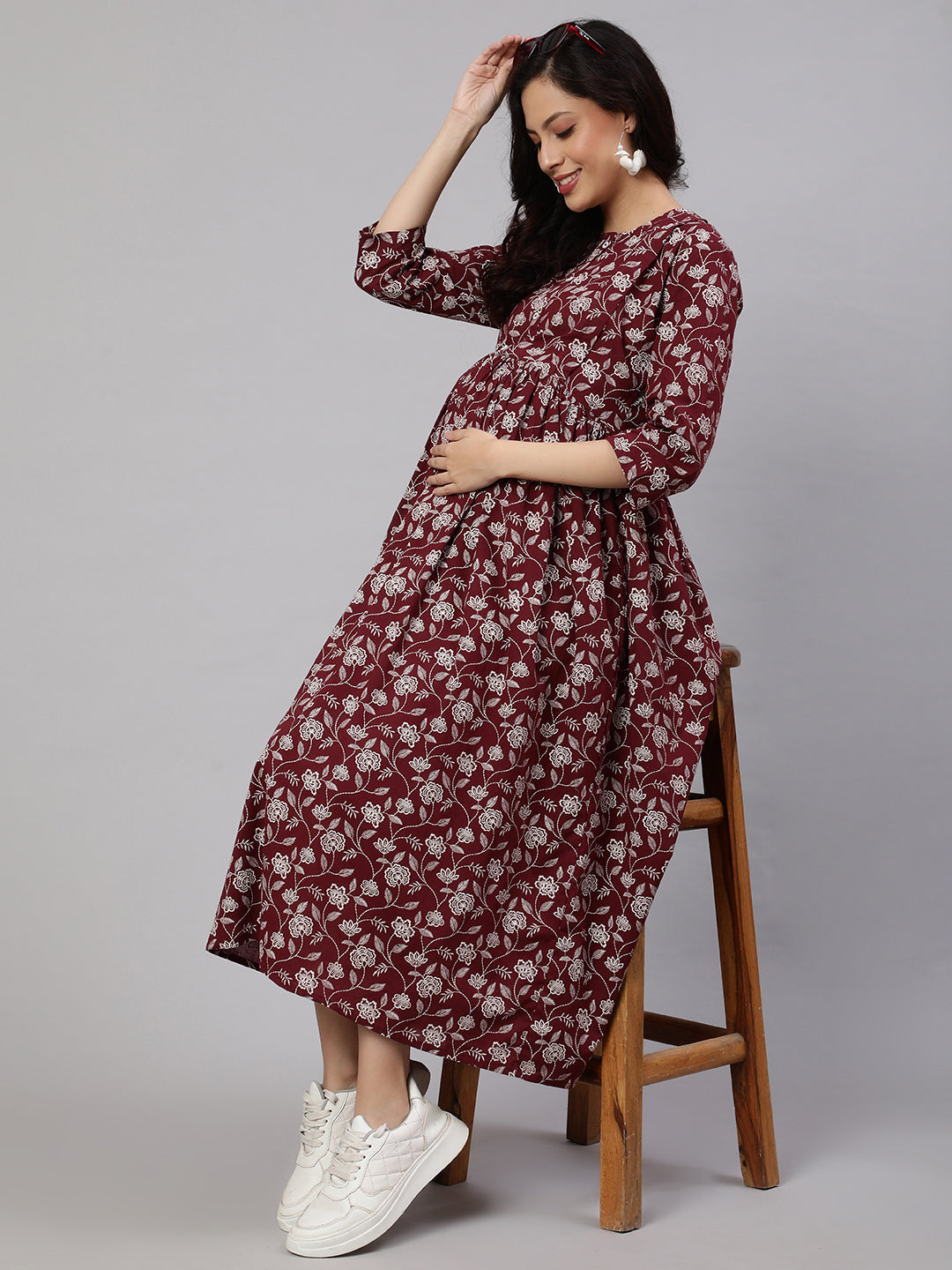In this professional portrait photograph, a pregnant woman is leaning against a high wooden stool. The background features a beige hue that complements the scene. She is elegantly dressed in a maroon dress adorned with white flowers, extending from her neck down to her ankles with three-fourths length sleeves. She wears white tennis shoes and large white earrings, along with red sunglasses perched on her black hair. Her right hand reaches towards her forehead, while her left hand tenderly cradles her belly, indicative of her pregnancy. Her gaze is cast downward with a gentle smile, encapsulating a serene and intimate moment. The composition suggests a posed setting, capturing the beauty and anticipation of impending motherhood.